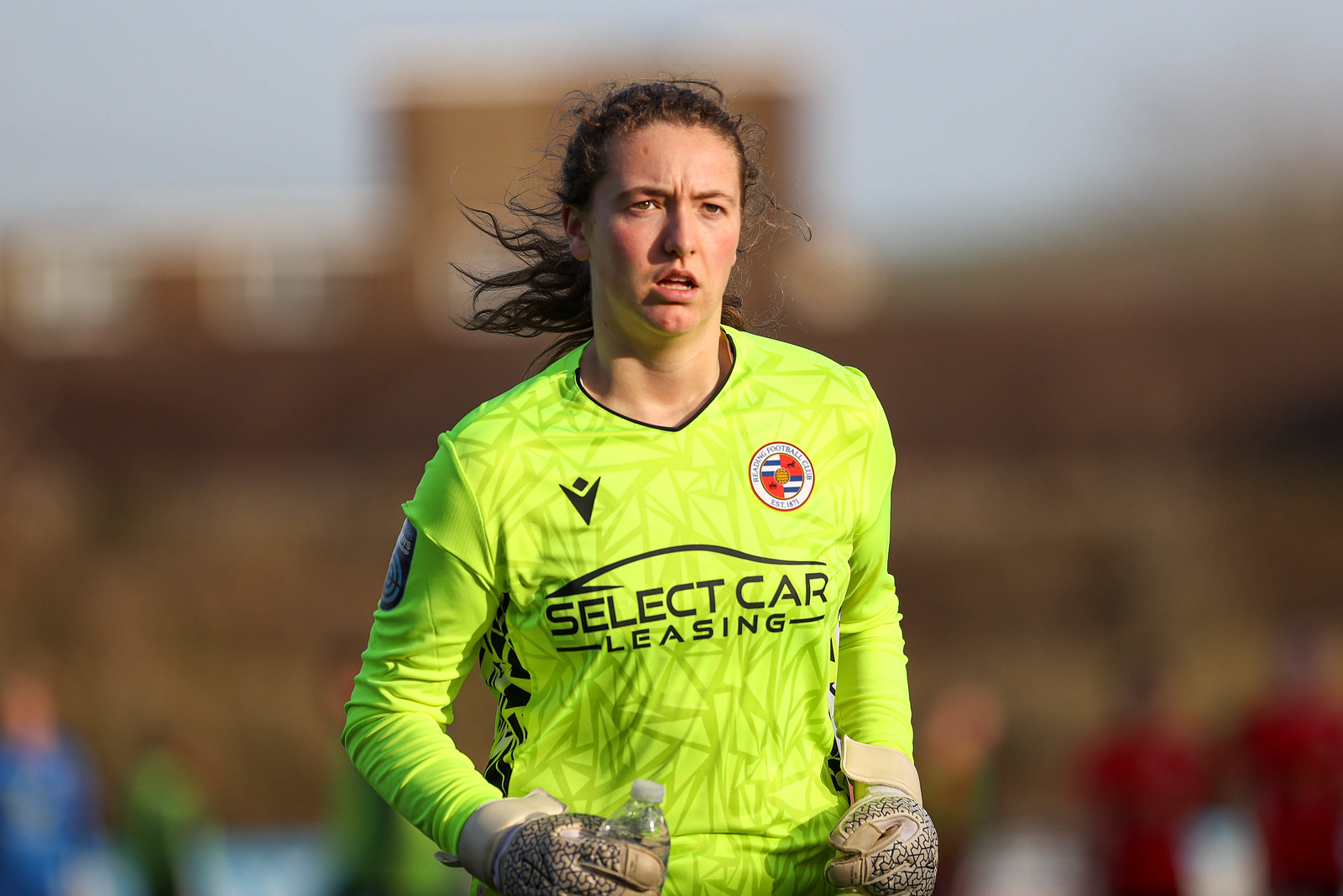This is a detailed photograph of a football goalkeeper, showing her face and upper body. She is adorned in a striking yellow, long-sleeve jersey emblazoned with "Select Car Leasing," along with several logos. Complementing her jersey are cream-colored, puffy gloves featuring a black design. With her mouth slightly open, she appears to be in motion, possibly walking or running, as evidenced by her frazzled hair blowing in the wind, which is tied up in a ponytail. Her cheeks are a rosy hue, suggesting she has been playing hard. In one hand, she holds a capped water bottle. The background is artistically blurred, highlighting a burst of colors: the sky's blue at the top, the likely brown hues of the stadium or its stands in the middle, and a mix of blue, green, and red at the bottom, likely representing the colors of other players' attire. Intriguingly, you can also discern blurred figures in red and blue shirts in the background, adding depth to the scene.